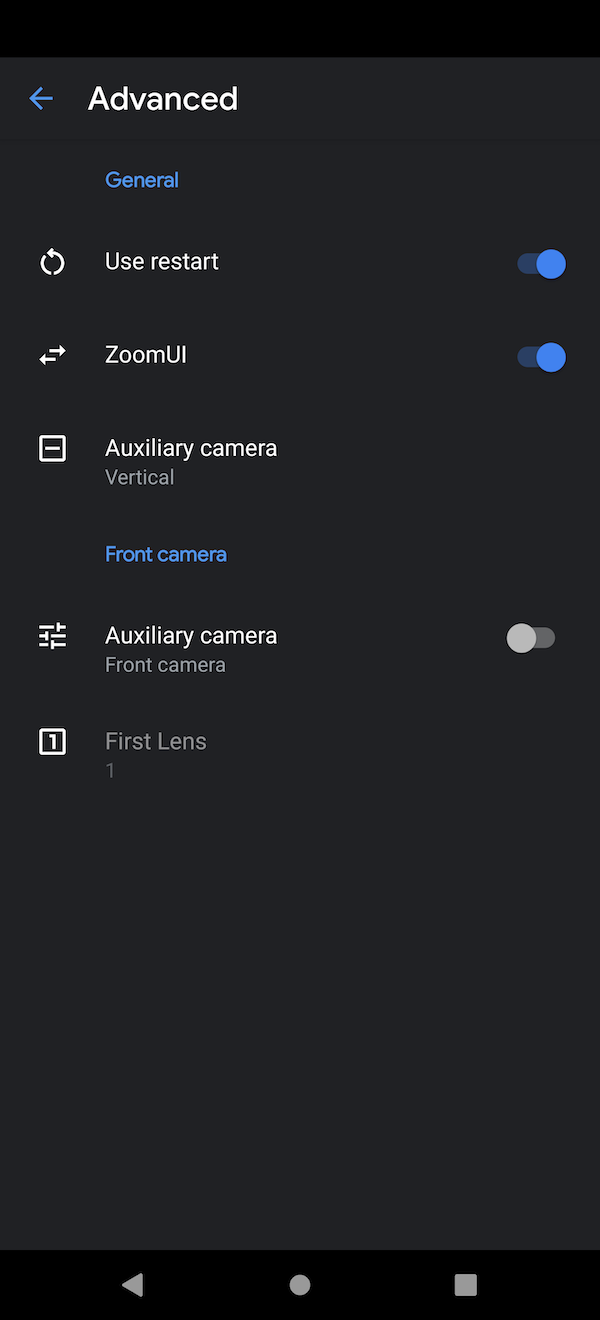This image is a screenshot of the "Advanced Settings" page from a mobile application. The background of the screenshot is black, with predominantly white text, while the actionable labels and buttons are accentuated in blue. At the top of the screen, there is no presence of a clock or time in the status bar; instead, it just features the word "Advanced" accompanied by a blue back arrow pointing to the left.

Below the "Advanced" title, the first section is labeled "General," displayed in blue text. The first option under this section features a refresh icon followed by the label "Use Restart," which has an associated toggle switch that is in the on position. 

Next, the "Zoom UI" option displays two stacked arrows pointing in opposite directions, with another toggle switch next to it, which is also switched on. 

Further down, the section labeled "Auxiliary Camera Vertical" includes the label "Front Camera" in blue text. Underneath, it states "Auxiliary Camera Front Camera" with a toggle switch to the right, which is currently turned off.

Lastly, the option labeled "First Lens" is mentioned at the bottom of the page, depicted in a grayed-out font, indicating that it is currently inactive or unavailable.